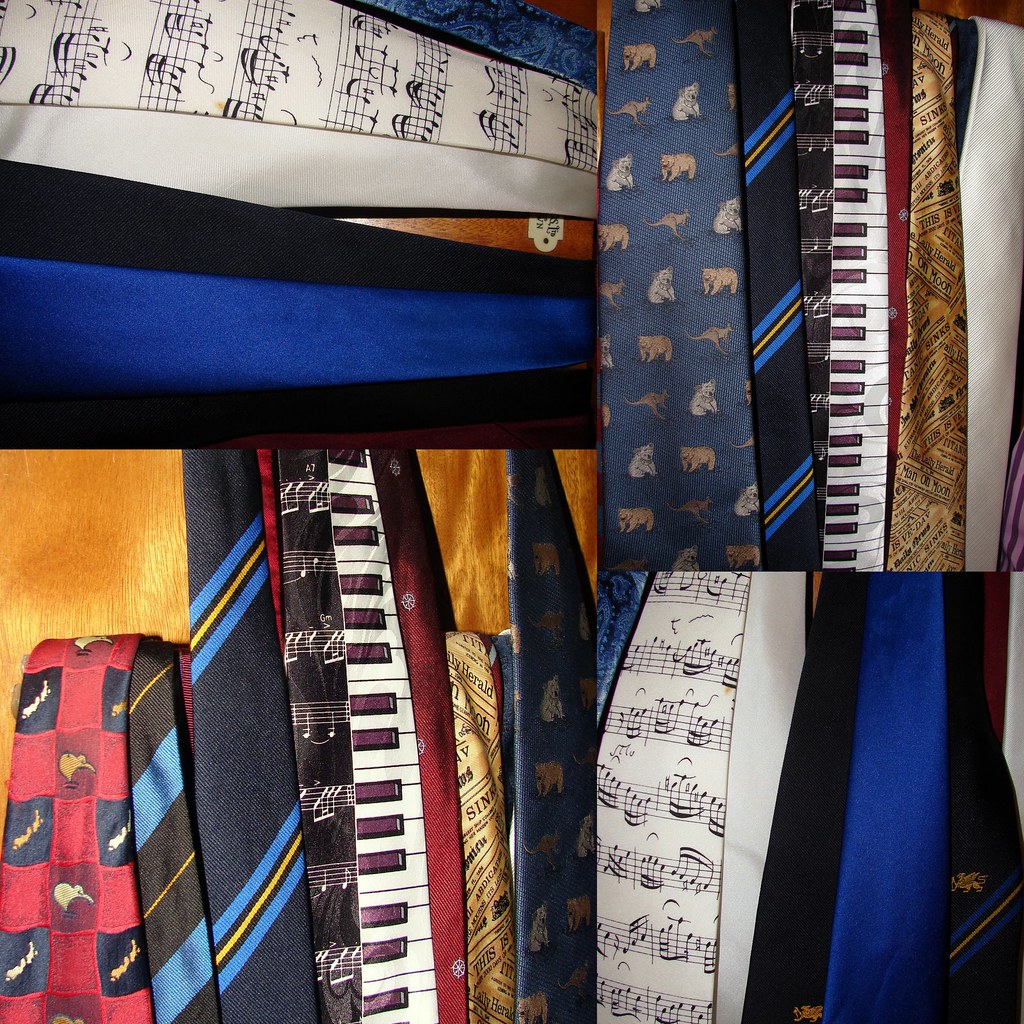This image is a detailed photo collage of various neckties, displayed across four segments. Each segment is meticulously organized, with two segments arranged horizontally and two vertically. At the top left, a collection of ties features a dark blue tie adorned with lighter blue and yellow stripes, a navy blue tie patterned with musical notes on a black background, a golden tie, and a tie with blue and white animal print showcasing dogs. In the top right, ties are presented against a darker backdrop, including a striking piano key tie set against a red background and a distinct gold tie adjacent to it. Moving to the bottom left, the ties are positioned vertically, with one red tie featuring a black checker pattern interspersed with images of birds in yellow and white. Another red tie incorporates piano keys along one side with musical notes scattered across another black tie. Lastly, a tie with diagonal blue and orange stripes is partially visible beneath a burgundy tie detailed with piano keys. The bottom right section mirrors the top layouts but transitions them vertically. Clearly, this collection highlights the owner's passion for music-themed ties while also showcasing an eclectic taste in patterned and novelty neckties, including a variety of plain and striped designs in various shades of blue, accentuating the diversity within their collection.